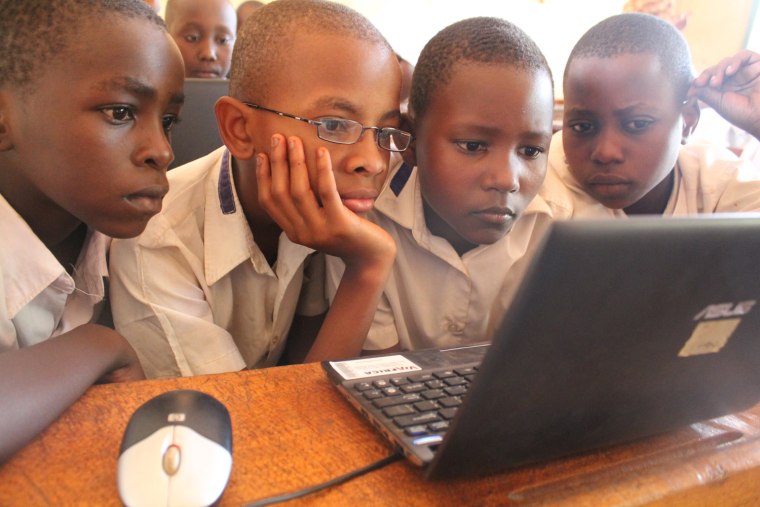This photo captures a group of six African school children, presumably ages 8 to 10, all with very short, closely shaved hair, huddled around a black Asus laptop positioned on the right side of a wooden desk. The four main children in the foreground are intently staring at the screen, their focus unwavering. Three additional children can be seen in the background, craning their necks to catch a glimpse of the laptop's display. All the children are dressed in white button-up shirts, consistent with a school uniform, and one child, second from the left, is distinctively wearing thin wire-frame glasses and resting his chin on his hand. The laptop is accompanied by a wired HP USB mouse on its left. The bright, sunny setting suggests they might be in a classroom. The scene is a moment of collaborative focus and curiosity, with the children gathered closely to engage with the content on the laptop screen.